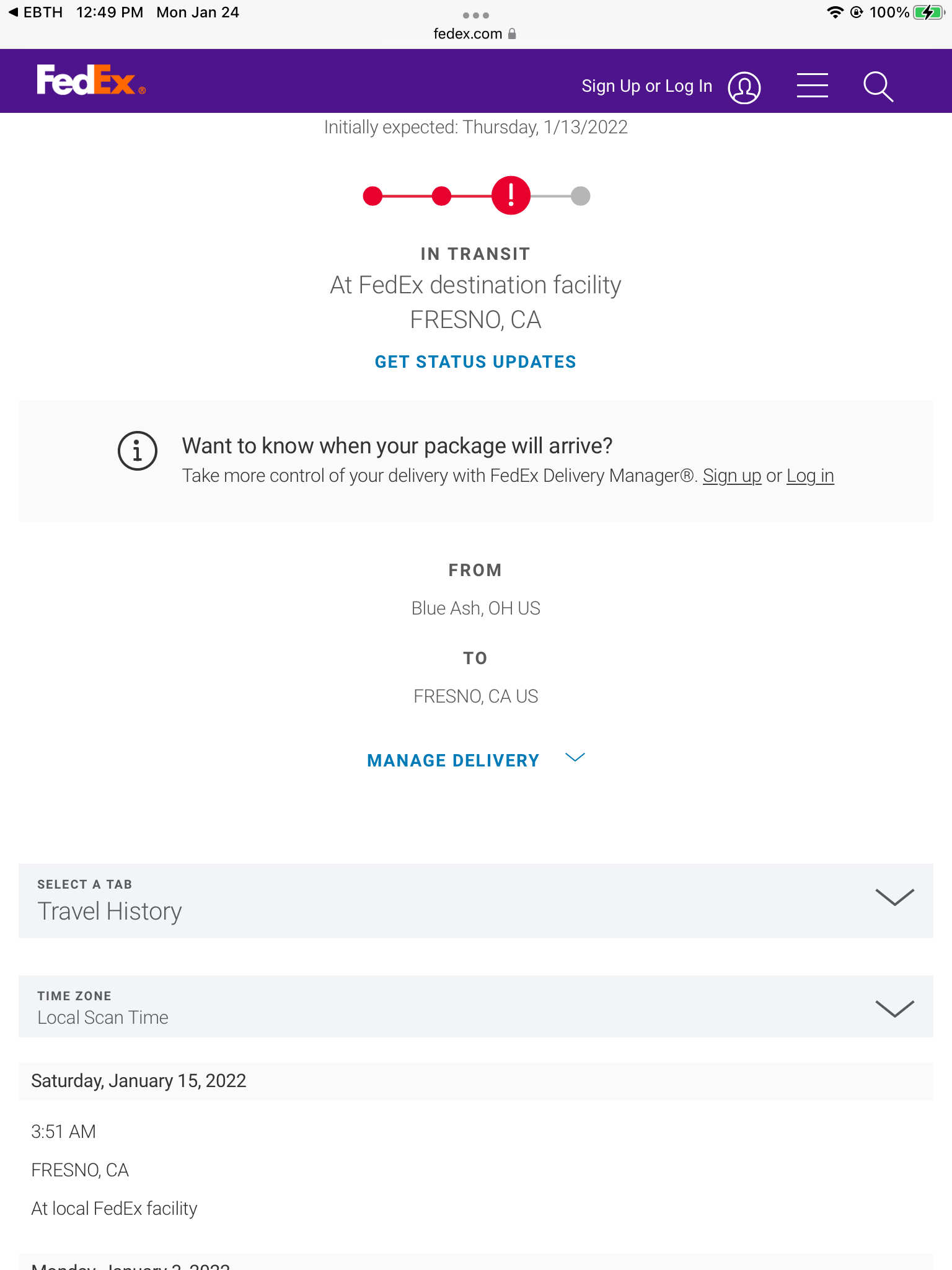This image is a detailed screenshot taken from the FedEx website, as indicated by the FedEx logo in the top left-hand corner, where "Fed" is in white and "Ex" is in orange. It appears to be captured from a mobile device, possibly a tablet or a smartphone. The screenshot represents a package tracking receipt, showing that the package is currently in transit. The estimated delivery date for the package is Thursday, January 13, 2022, and it is destined for Fresno, California, traveling from Ohio. 

The package's transit status is prominently displayed at the top. Below, additional details regarding the package's current location and destination are provided. In the center of the screen, a blue-colored "Manage Delivery" option is available for the user to interact with. 

The top right-hand corner of the device interface shows a full battery charge at 100%. Meanwhile, the top left-hand corner displays the current time as 12:49 PM and the date as Monday, January 24.